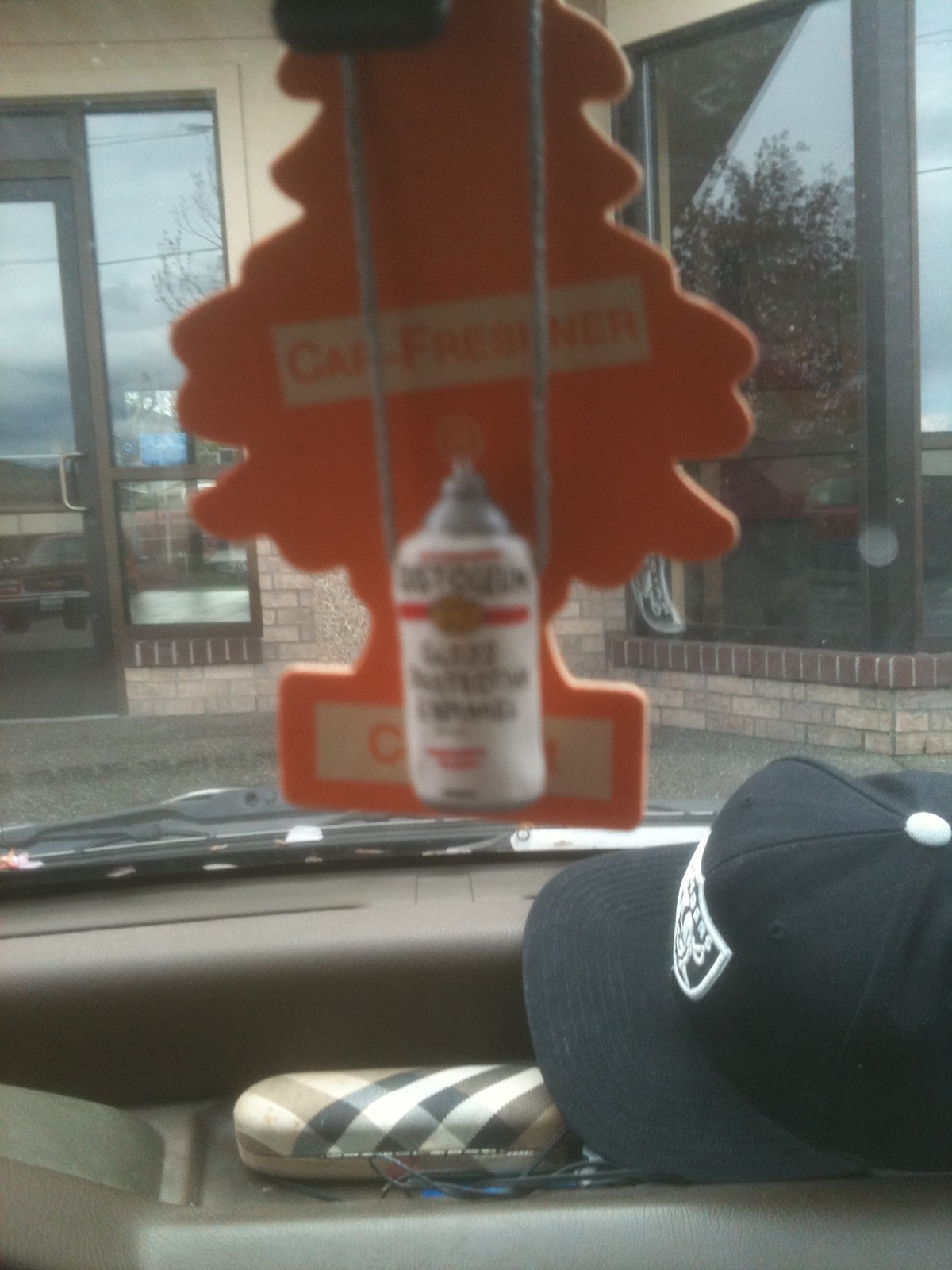The image captures the view from inside a car, focusing through the front windshield towards the exterior of a store. A scene unfolds featuring a light grey brick wall and a door on the left, distinguished by its gold handle and central glass pane. Adjacent to the door is a clear window, while to the right, a larger rectangular window with rounded edges peeks into view, segmented by wooden columns. Dominating the foreground is a red, tree-shaped air freshener with white text, suspended from the rear-view mirror. Below, the car's standard dashboard is partially occupied by items: a black baseball cap with a white logo and button, facing left, and a plaid glasses case in shades of cream, dark brown, black, and white. The air freshener also seems to have a spray paint can element hanging below it, adding to the assortment of items seen inside the vehicle.